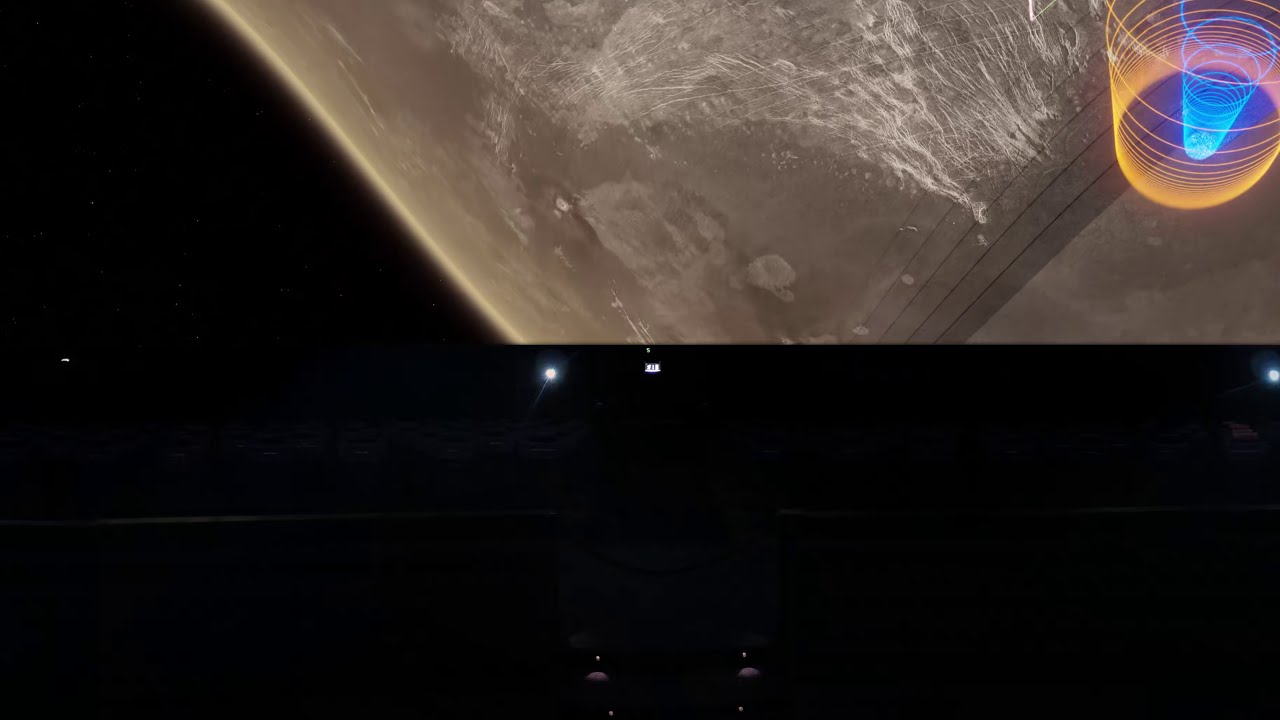The image captures the interior of a large movie theater, observed from above in a dimly lit room. Dominating the scene is an enormous screen displaying a beige or grayish planet with a thin atmosphere set against a dark backdrop of space. The planet features a diagonal line and some visible craters and marks on its surface. The top right corner of the image showcases a complex pattern of circular and spiral shapes in oranges and neon blues, interspersed with black stripes, which appear to overlay the main planetary image.

In the bottom left corner of the frame, an illuminated exit sign confirms the setting as a cinema. Additionally, there are several other lights around the screen, particularly noticeable along the floor on the right and left sides. The lower half of the image is quite dark, obscuring the view of the auditorium, although a few seats can be partially discerned, reinforcing the identification of this space as a movie theater.